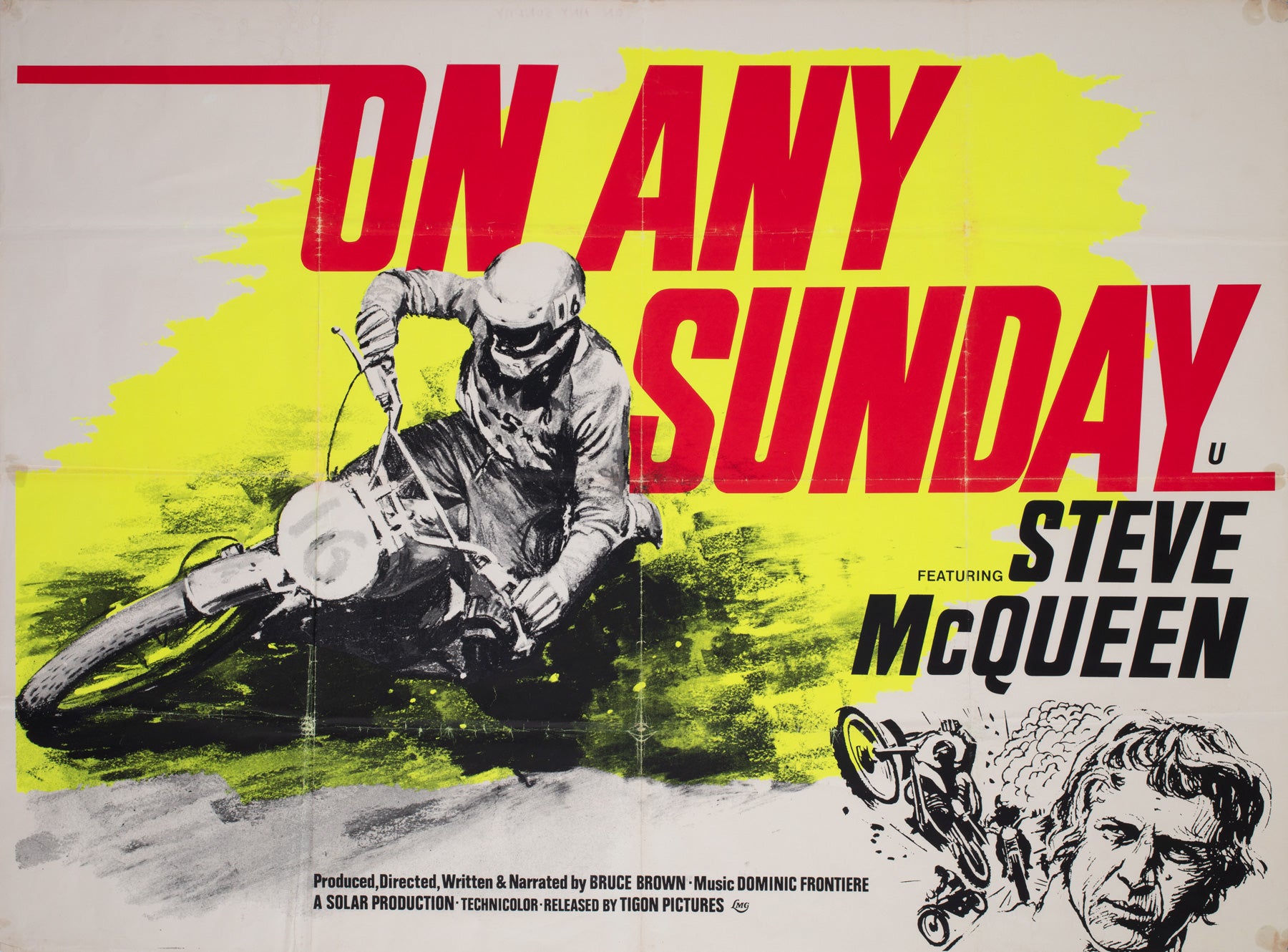The poster for the movie "On Any Sunday" prominently features a striking yellow background with a black and white illustration of a man riding a motorcycle, likely Steve McQueen, who is facing left. The rider is wearing a helmet marked with the number 16 and appears to have his sleeves rolled up. The title, "On Any Sunday," is boldly written in red at the top and on the right side of the image. Below the word "Sunday," the text reads "Featuring Steve McQueen." At the bottom right of the poster, additional images include a man's head and several motorcycles seemingly escaping from an explosion. The bottom of the poster credits Bruce Brown as the producer, director, writer, and narrator, with music by Dominic Frontier, and notes that it is a Solar Productions film. The overall color scheme includes reds, yellows, grayish whites, and blacks, contributing to the intense and dynamic feel of the poster.